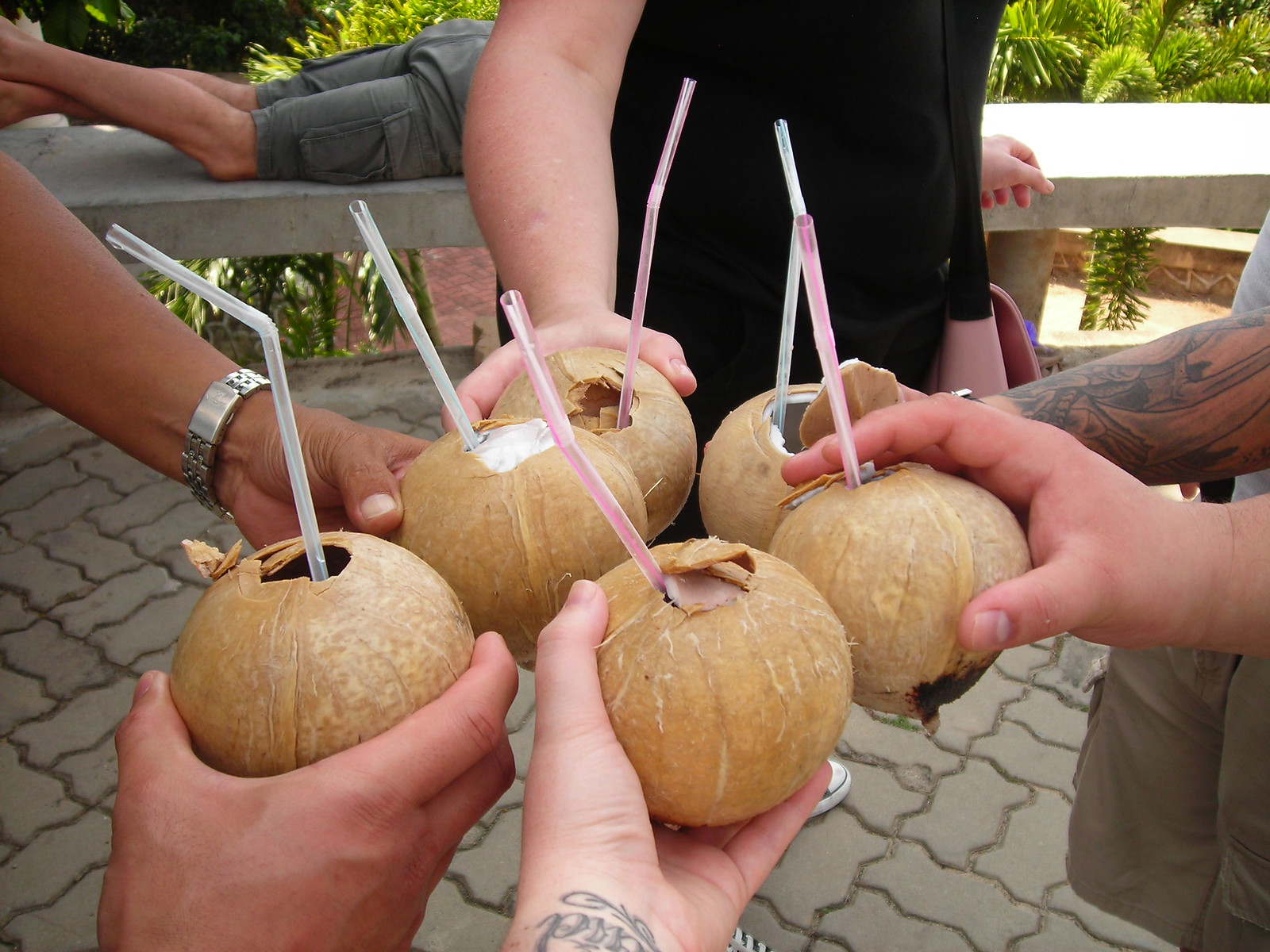The close-up photo centers on six hands holding small, round coconuts in a celebratory toast. The coconuts have been shaved into smooth spheres, each fitted with colorful straws, primarily pink and clear. The background reveals a decorative gray brick surface and a concrete bench. A person in gray shorts lies stomach-down on the bench, with legs playfully crossed behind them. Among the hands holding the coconuts, two are adorned with tattoos and one sports a silver watch. Surrounding this scene, tall palm-like trees accentuate the tropical atmosphere.